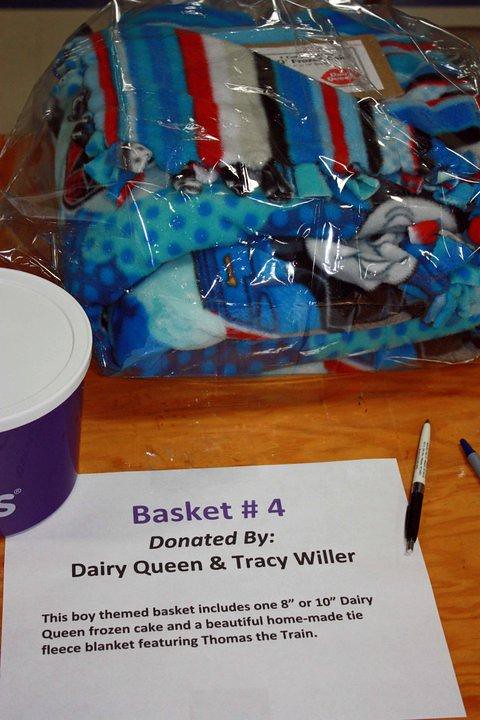This image shows a detailed display likely set up for a fundraising event or silent auction. Central to the photograph is a piece of paper on a wooden table, which is held down by a round, purple container that appears to be an ice cream tub. On top of the tub is a plastic bag containing a beautifully homemade tie fleece blanket featuring Thomas the Train. The paper has bold text reading "Basket #4," with details indicating it is "Donated by Dairy Queen and Tracy Willer." The description further explains that this boy-themed basket includes one eight-inch or ten-inch Dairy Queen frozen cake and the Thomas the Train blanket. Adding to the setup, there are two pens positioned to the right of the paper. Upon closer inspection, a coupon from Dairy Queen is also visible within the plastic-wrapped blanket.